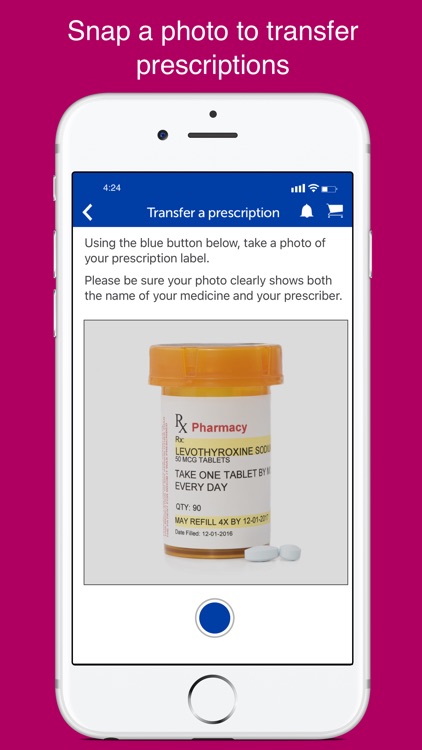Screenshot Description: 

The image displays a screenshot of a prescription drug transfer application, framed within the interface of a simulated phone emulator. The emulator itself is placed atop a vivid red rectangle. At the top of the rectangle, bold white text clearly states, "Snap a photo to transfer prescriptions."

Within the emulator, the main screen is dominated by a blue button labeled "Transfer Prescription." Below this button, a concise set of instructions guides the user on the steps required to transfer a prescription.

Prominently featured in the middle of the screen is a detailed photograph of a prescription bottle, viewed head-on. The pharmacy label on the bottle is distinctly visible, showcasing the following details: the highlighted name of the medication, its dosage, clear instructions on how to take the medication, the total quantity of pills, and the number of refills available. To the right of the bottle, a few loose pills are displayed, emphasizing the medication context.

Beneath the photograph, another blue button instructs the user to "Take a picture," signaling the next step in the prescription transfer process. The screenshot concludes at this point, just above the bottom edge of the phone emulator.